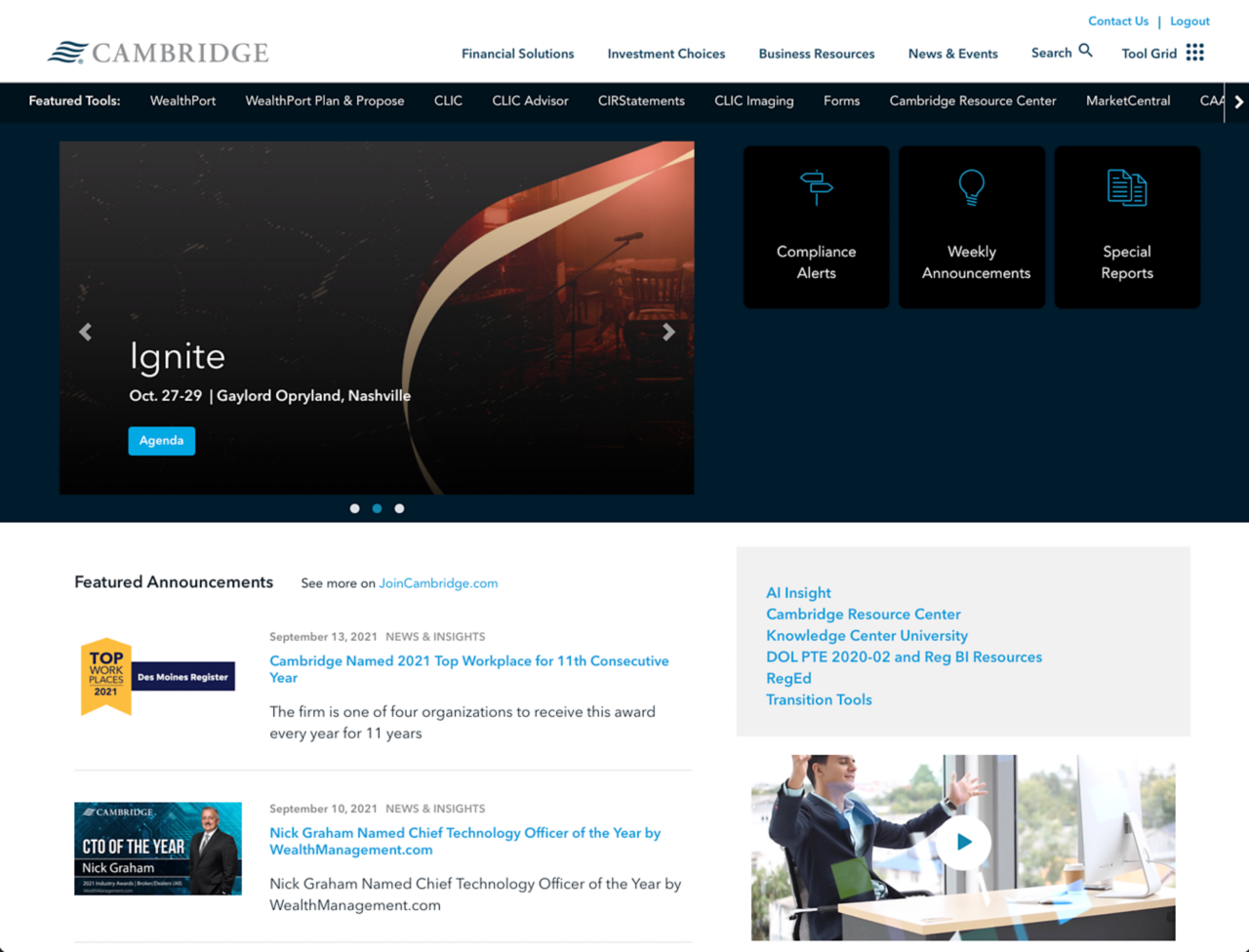**Caption:**

The screenshot features the homepage of the investment firm, Cambridge, highlighted at the top left corner in all capital letters. Spanning across the top of the page, various navigation options are visible, including "Financial Solutions," "Investment Choices," "Business Resources," "News and Events," "Search," and "Tool Grid." Below this, set against a black background, is another row of navigation links: "Featured Tools," "WealthPort," "WealthPort Plan and Propose," "CLIC," "CLIC Advisor," "CIR Statements," "CLIC Imaging," "Forms," "Cambridge Resource Center," and "Market Central." The subsequent line includes options for "Compliance Alerts," "Weekly Announcements," and "Special Reports."

On the left side of the page, larger text announces the "Ignite" event, scheduled for October 27-29 at Gaylord Opryland in Nashville. There is a slightly blurry image accompanying this text, depicting a room with a microphone and some chairs. Beneath this event notice, there is a section for featured announcements, celebrating Cambridge being named a "Top Workplace" by the Des Moines Register for the 11th consecutive year in 2021.

Further down is a professional photo of a man in a business suit with the caption recognizing Nick Graham as the "CTO of the Year," awarded by WealthManagement.com. To the right, detailed information about the firm's location is noted. Beneath that, another image shows a man in a business suit standing near a desk.